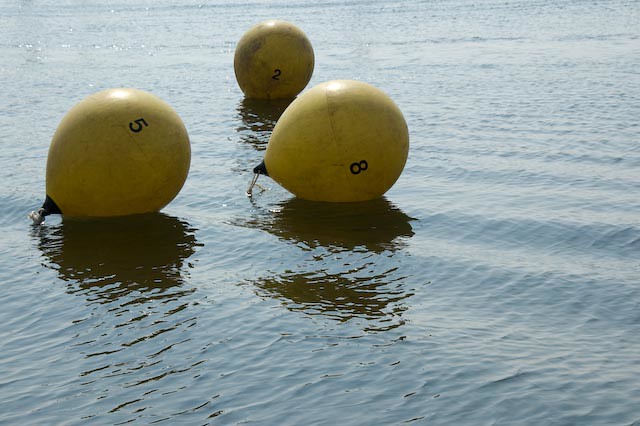This photograph depicts a serene body of water, possibly a lake or a calm ocean, with three yellow buoys floating on its surface. The buoys are weathered and bear visible signs of prolonged exposure to the elements, such as dirt and debris. Each buoy is marked with a distinct number: 5, 8, and 2. The buoys are arranged with numbers 5 and 8 in the front, side by side, and number 2 slightly behind them, partially submerged. They appear to be tethered to something below the water’s surface via visible ropes. The water is tranquil with only faint ripples, and the scene suggests a sunny day, as indicated by the shadows cast on the water. The entire background is filled with the still, blue expanse of the water, with no sky or other elements in view. The buoy marked with the number 5 is situated on the far left, 8 to its immediate right, and 2 is positioned further back, between the other two.